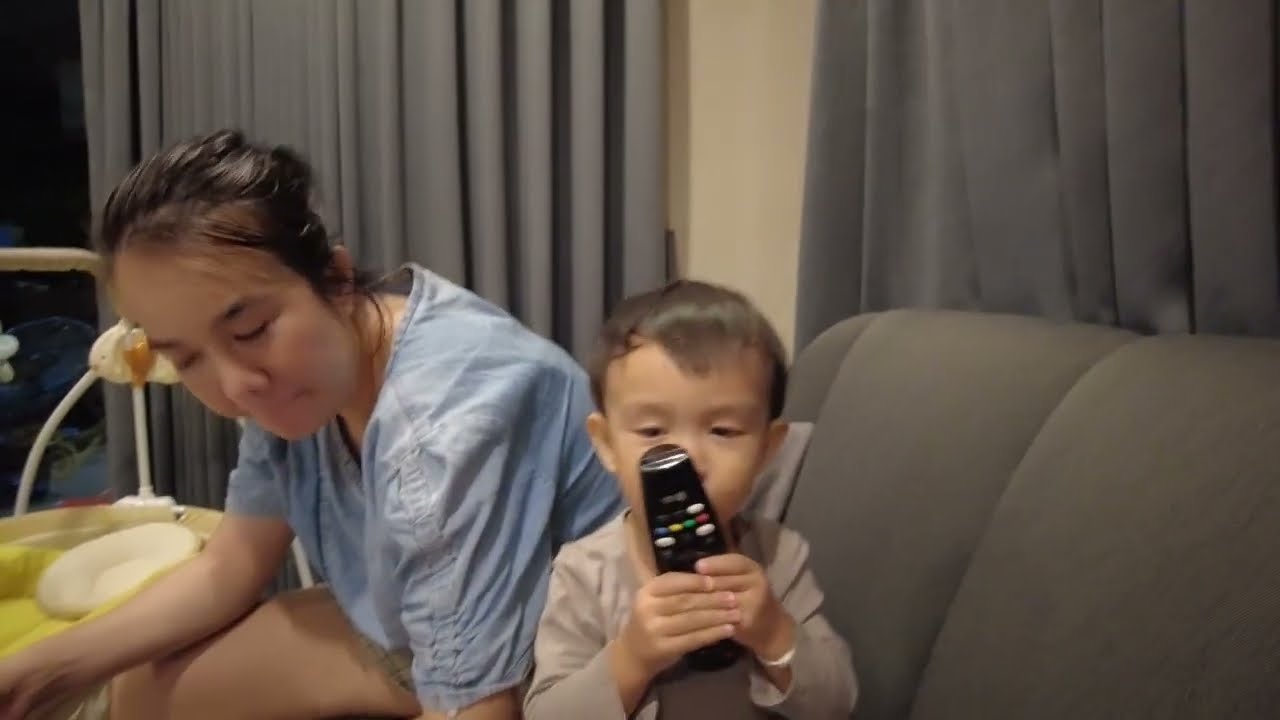The photograph captures a tender, casual moment between a small East Asian boy and what appears to be his mother, both seated on a dark gray couch. The boy, who looks to be about two years old, is positioned on the right-hand side of the image, holding a remote control tightly in both hands, although it's clasped backwards so that he is looking at the battery compartment. He has black, somewhat messy hair and is dressed in a tan long-sleeved shirt. 

Beside him, his mother, also of East Asian descent, is slightly bent over, possibly about to get up. She is wearing a light blue top that resembles a nurse's gown, and her dark hair is pulled back into a messy bun. Her eyes are closed and her head is tilted to the side, giving the impression she might be blinking or resting momentarily. 

To her right, an empty plate rests on a nearby table. Behind them, two windows are adorned with light gray drapes against a beige wall. Additionally, a baby accessory, which looks like a "sit and spin" or baby walker with rattles, is visible in the background, contributing to the family atmosphere.